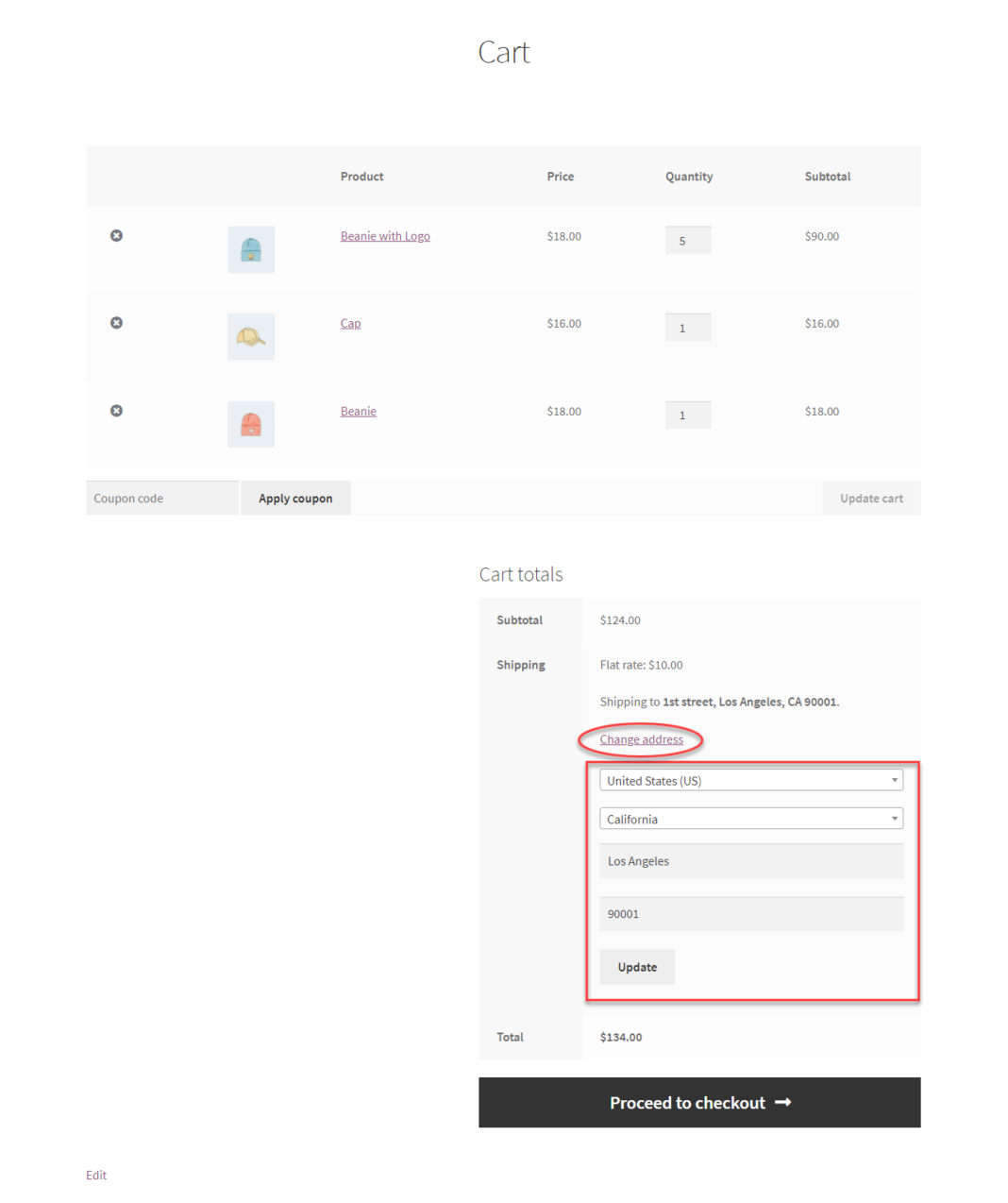Here is a detailed, cleaned-up caption based on the given audio description:

---

The image depicts a detailed shopping cart interface on a webpage with a gray background and black text. The cart is displayed in a table format with four columns labeled "Products," "Price," "Quantity," and "Subtotal." 

- **Products:**
  1. Beanie with Logo (blue)
  2. Cap (yellow)
  3. Beanie (red)

- **Prices:**
  - Beanie with Logo: $18 
  - Cap: $16 
  - Beanie: $18

- **Quantities:**
  - Beanie with Logo: 5
  - Cap: 1
  - Beanie: 1

- **Subtotals:**
  - Beanie with Logo: $90 (calculated as $18 x 5)
  - Cap: $16
  - Beanie: $18
  - Total number of items: 7
 
At the bottom left, there's a section for entering a coupon code, consisting of a text box with a placeholder labeled "Coupon Code," and an adjacent button labeled "Apply Coupon," both in gray with bold black text.

On the bottom right, there's a "Update Cart" button, also in gray with black text.

Below this, a section on the right half of the screen features:
- **Subtotal:** $124
- **Shipping:** Flat rate of $10
  - Shipping to: 1st Street, Los Angeles, CA, 90001
  - Address fields are outlined in red to indicate they are selected.
  - Country: United States (selected from a dropdown)
  - State: California (selected from a dropdown)
  - City: Los Angeles (in a text box)
  - ZIP Code: 90001 (in a text box)
  - An "Update" button in gray with black text for updating the address.

At the very bottom, it lists:
- **Total:** $134
- A prominent black button with white text that says "Proceed to Checkout," accompanied by a right-pointing arrow.

---

This revised caption provides a clear and detailed description of the shopping cart interface, describing both the visual layout and the detailed content of each section.